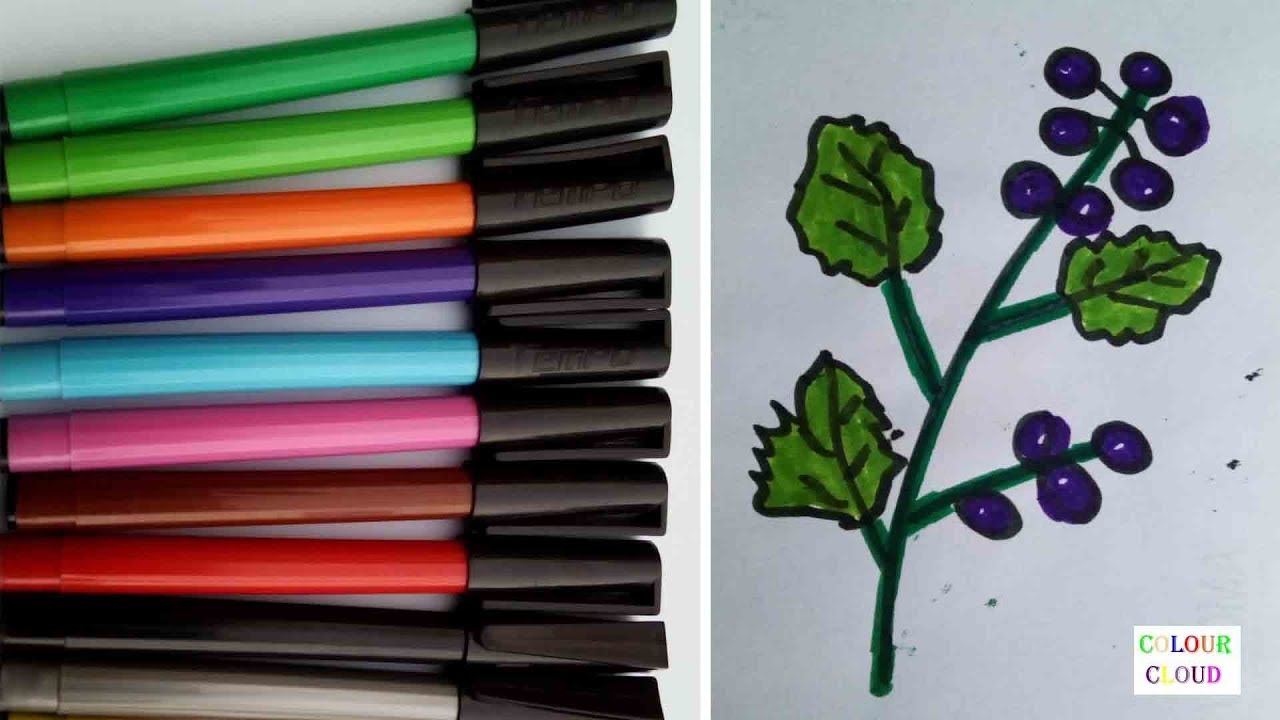This image is a split advertisement showcasing a set of colorful markers and a drawing made with them. On the left side, there is a neatly arranged row of markers, each featuring a black cap. The colors of the markers, starting from the top, include two shades of green, orange, purple, light blue, pink, copper, red, and black. The right side displays a doodle of a fruiting plant with a stem, a couple of green leaves, and clusters of round, blue berries. The outlines of the plant and berries are drawn in black, demonstrating the marker's precision. The background is blue, and a logo reading "Color Cloud" is positioned at the bottom right, indicating the company's name. The drawing illustrates the vibrant and diverse colors these markers can produce.